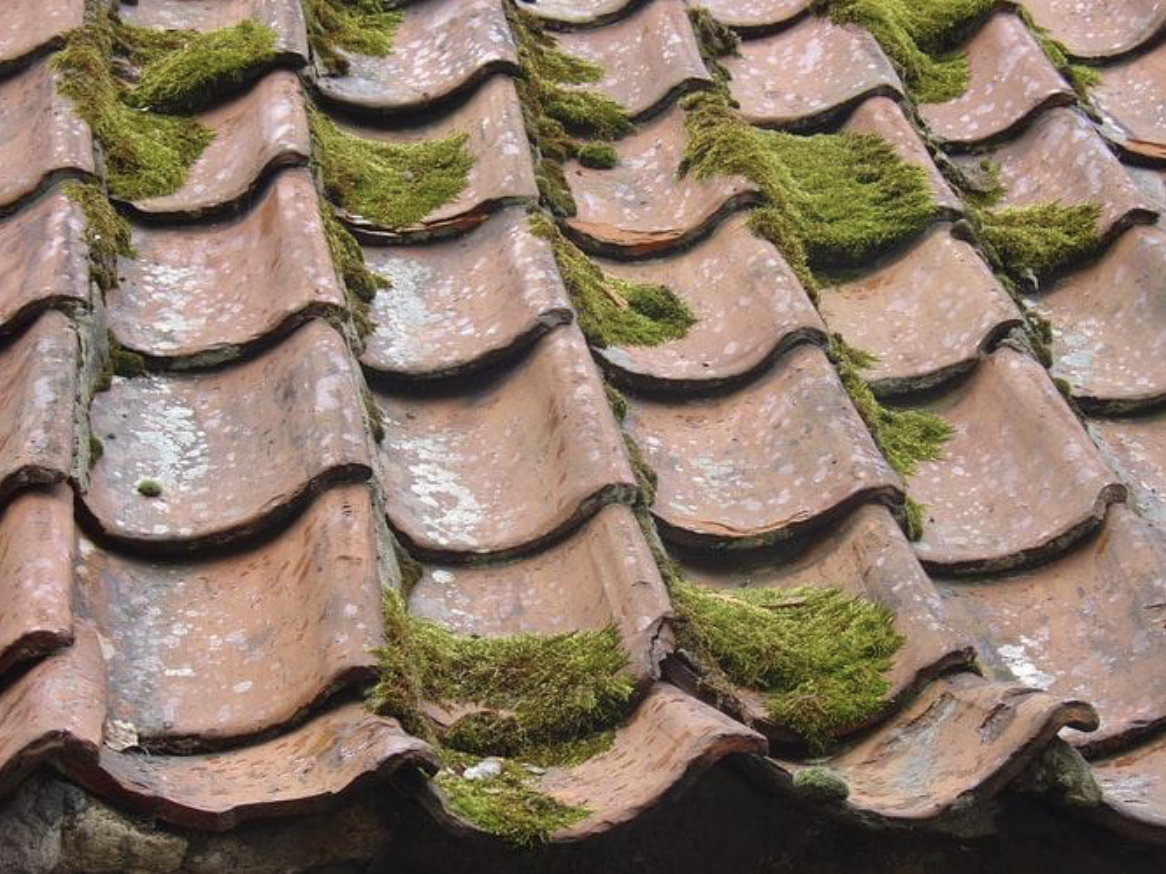The image captures a close-up view of an old, weathered terracotta roof in daylight. The overlapping, wave-shaped tiles exhibit a reddish-orange hue characteristic of traditional Spanish clay roofing. Upon closer inspection, the tiles show signs of significant wear and aging, marked by chips, white speckled discoloration, and areas where the coloration has faded due to exposure to the elements. Green moss grows sporadically across the roof, further indicating its long-standing neglect and lack of maintenance. On the left, the roof slopes downward toward the edge, revealing a small portion of the underlying stone structure of the building, hinting at its antiquated state and urgent need for repair.